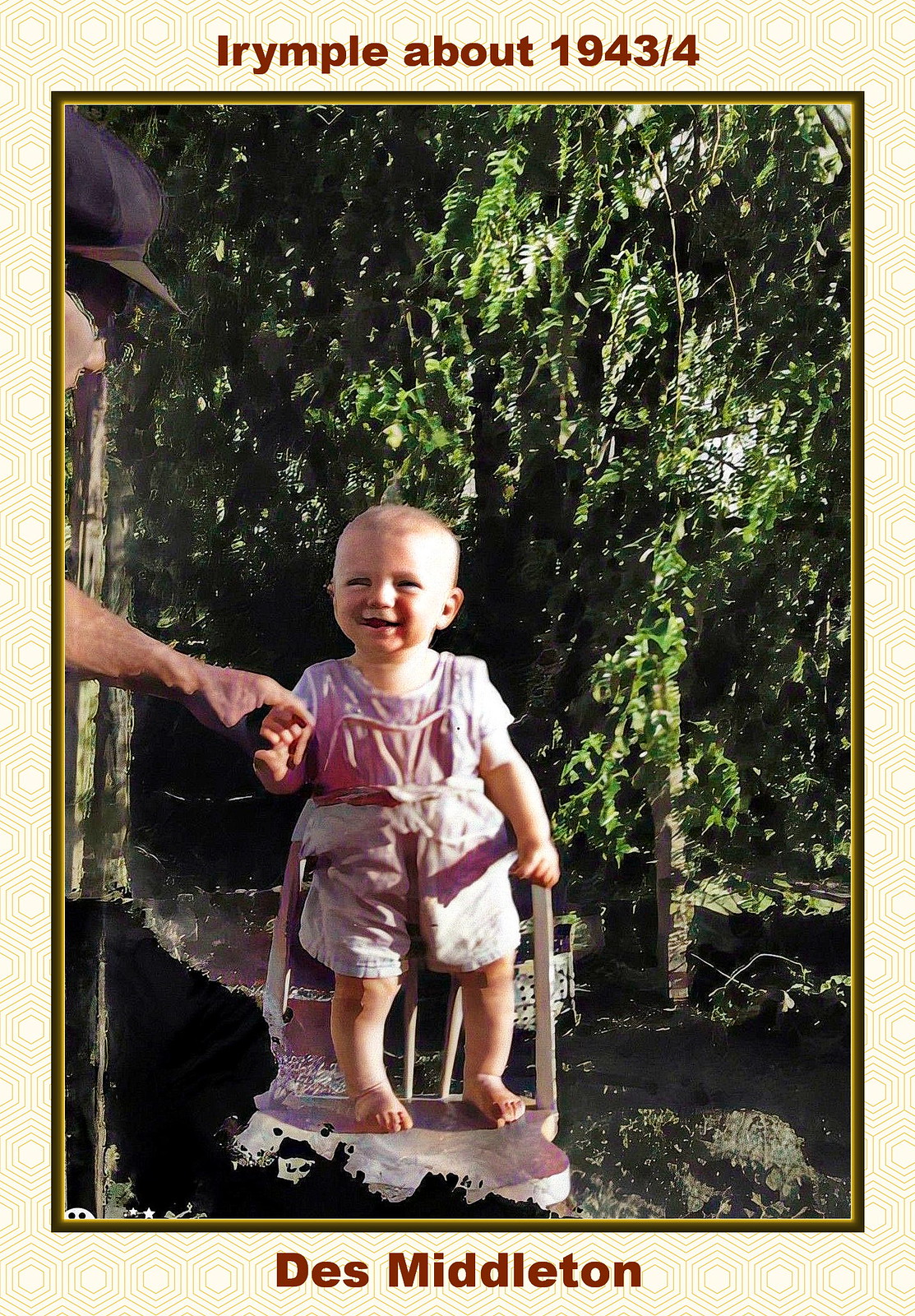This vertical photo, framed by a light yellow border with hexagon patterns, features a smiling baby standing barefoot on a slightly elevated, raggedy chair. The baby, wearing a pink undershirt and white and pink shorts, grasps the hand of an off-camera man whose arm extends from the center left of the image. In the background, there is a large green tree with thick foliage and a visible trunk to the right, set against a ground of dark dirt with hints of grass. Above the photo, brown text on a white background reads "Erin Poole about 1943/4," while the bottom of the photo similarly notes "Des Middleton" in brown text. A subtle filter over the image adds a vintage, slightly faded feel to the scene.